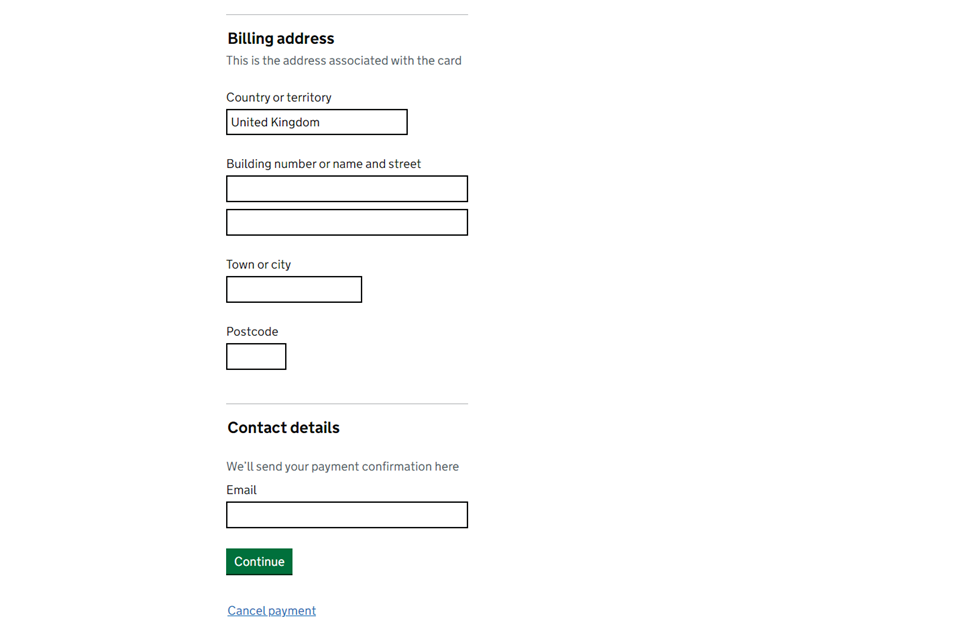The image depicts a page in an online purchase process where you must enter your billing address. At the top, there is a heading that indicates this is the address associated with your card. The first subsection, labeled "Country or Territory," is already filled in with "United Kingdom." Below this, there are two input fields labeled "Building Number or Name" and "Street" for you to enter the relevant details. Further down, there are additional fields for "Town or City" and "Postcode." 

Next, there is a section titled "Contact Details," which contains a field where you must input your email address, accompanied by a note stating that the payment confirmation will be sent to this email. At the bottom of the page, a prominent green "Continue" button with white text is noticeable, designed to stand out against the rest of the page. Below this button, there is a smaller blue section with a "Cancel Payment" button, which allows you to exit the process if you change your mind.